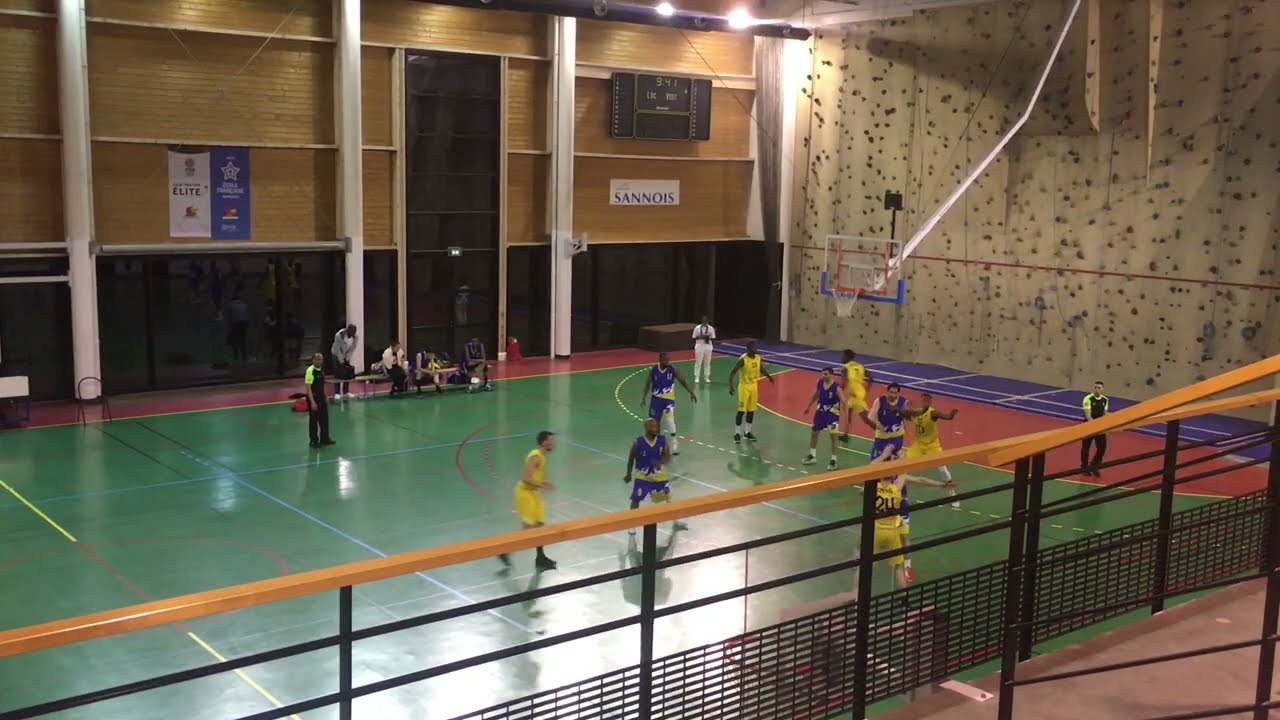This is a detailed photograph of an indoor basketball court, capturing a competitive match between two men's teams donning yellow and blue jerseys. The action is concentrated on the right side of the green court, which features a red innermost circle surrounding the basket. Visible in the background is a beige wall adorned with dark gray spots. Prominently displayed above the scene, a scoreboard reads "9 4 1" and is flanked by two banners: one on the right side saying "SANNOIS" in blue font and another on the left marked "Elite." The gymnasium is well-illuminated, with overhead lights casting a bright glow on the court. Black glass windows or screens surround the space, providing reflections of the players and spectators. Beneath these windows and near the right side of the court, there is a climbing wall visible behind the basketball hoop. Support staff and other athletes are seen walking around or sitting on benches. Various elements like railings, pillars, and possibly a referee on the top left, add to the busy atmosphere of this indoor venue. The photo appears to be taken from an elevated position in the bleachers, giving an overall view of the energized and well-attended event.